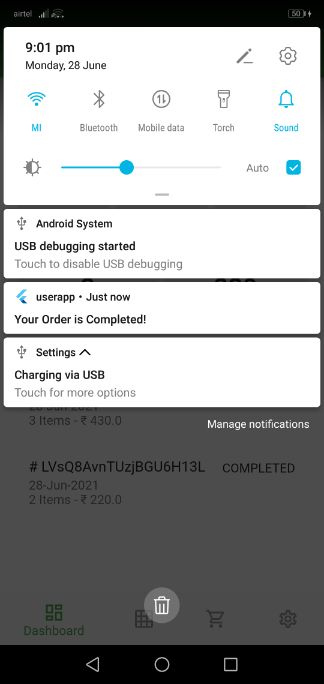The screenshot displays a segment of a smartphone's interface taken on Monday, June 28, at 9:01 p.m. At the top of the screen is a white rectangular box showing the date and time. To the right of this box are two icons: a pencil icon followed by a gear icon. Below these, various connectivity icons are visible. From left to right, they include a blue Wi-Fi signal icon, a Bluetooth signal icon, a mobile data indicator, a torch icon, and a bell icon labeled "Sound."

Below these, there is a brightness adjustment slider with an indicator to allow users to modify the screen's brightness. Underneath this slider, a notification from the Android system states "USB debugging started," with an instruction to "Touch to disable USB debugging." Directly under this notification is another box that states "User app just now. Your order is completed." Finally, at the bottom of the screenshot, there is a notification from the settings labeled "Charging via USB. Touch for more options."